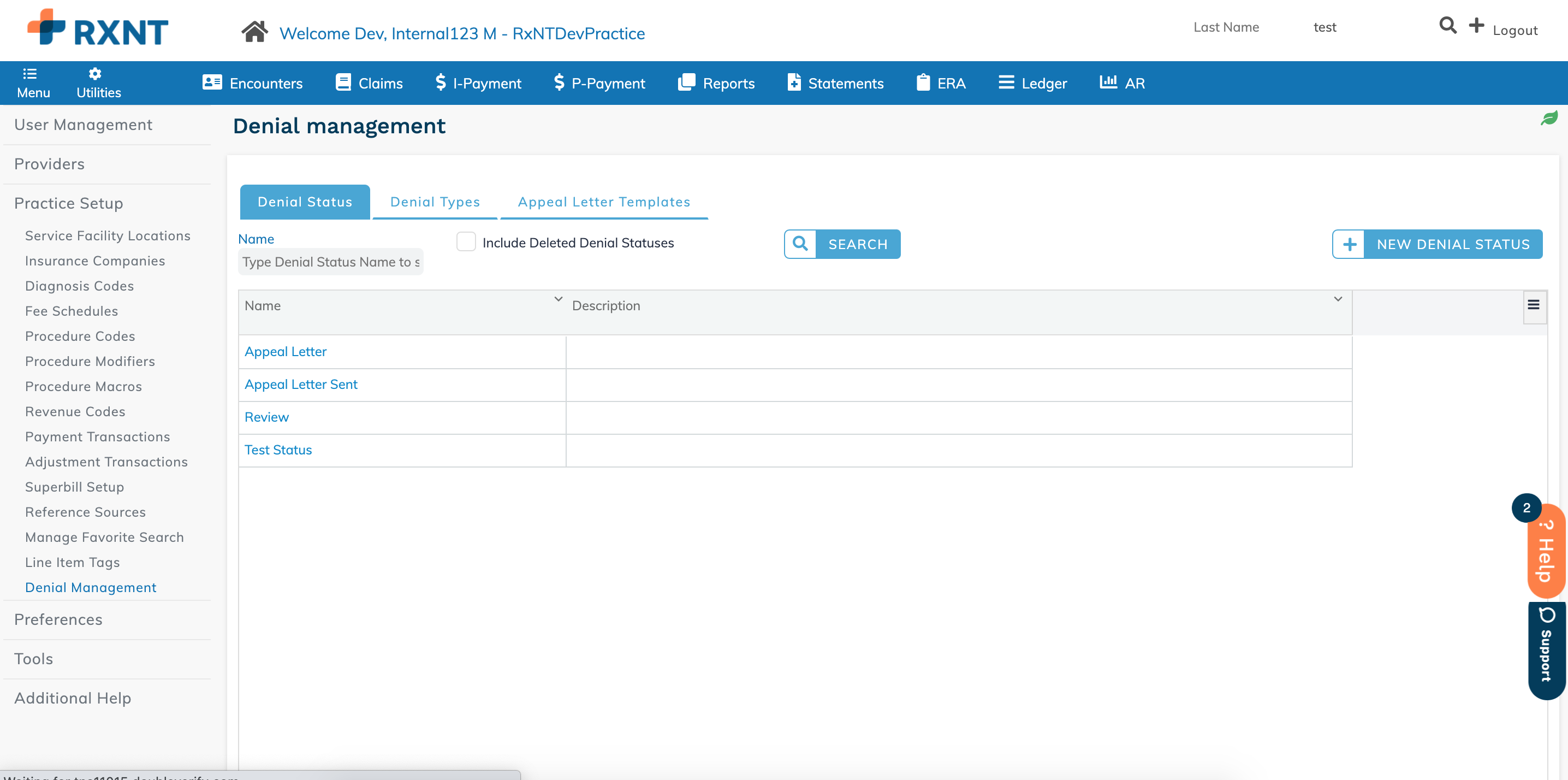**Detailed Caption:**

This screenshot showcases the RXNT medical practice management software interface. At the top-left corner, adjacent to the all-capitalized blue "RXNT" logo, there's a distinctive plus sign. The plus sign features two upper segments in orange and two lower segments in blue, all of which curve gracefully towards one another. The segments on each side curve inward, creating a sharp contrast between opposite segments.

To the right of the logo, there is a home button and a welcoming message stating "Welcome dev internal123m-rxnt dev practice." Following this message, there's a search bar with icons indicating functionalities like 'Last Name', 'Test', and a magnifying glass. Additionally, there's a 'Logout' button.

Below this, on a blue menu bar, the interface lists various options: 'Utilities', 'Encounters', 'Claims', 'IA-Payment (with a dollar sign)', 'P-Payment (with a dollar sign)', 'Reports', 'Statements', 'ERA', 'Ledger', and 'A/R'.

The left side of the interface features an extensive vertical menu. Key categories include 'User Management', 'Providers', 'Practice Setup'—which further expands into submenus like 'Service Facility Locations', 'Insurance Companies', 'Diagnosis Codes', and others. Under this main menu, there are additional options such as 'Preferences', 'Tools', 'Additional Help', with approximately 15 submenus in total.

Specifically highlighted in the submenu under 'Practice Setup' is 'Denial Management'. This section contains three tabs: 'Denial Status', 'Denial Types', and 'Appeal Letter Templates', with 'Denial Status' being the current selection. The 'Denial Status' tab provides columns labeled 'Name', 'Denial Status Name 2', 'Name Description', 'Appeal Letter', 'Appeal Letter Sent', 'Review', and 'Test Status'. There is also a search bar on the right side of this section, with a 'Plus' button for new entries and a button labeled 'New Denial Status'.

This interface appears to be a feature-rich, highly detailed tool for managing multiple aspects of a medical practice, from patient encounters and claims to denial management and reporting, although the actual use and functionality may require further user familiarity.